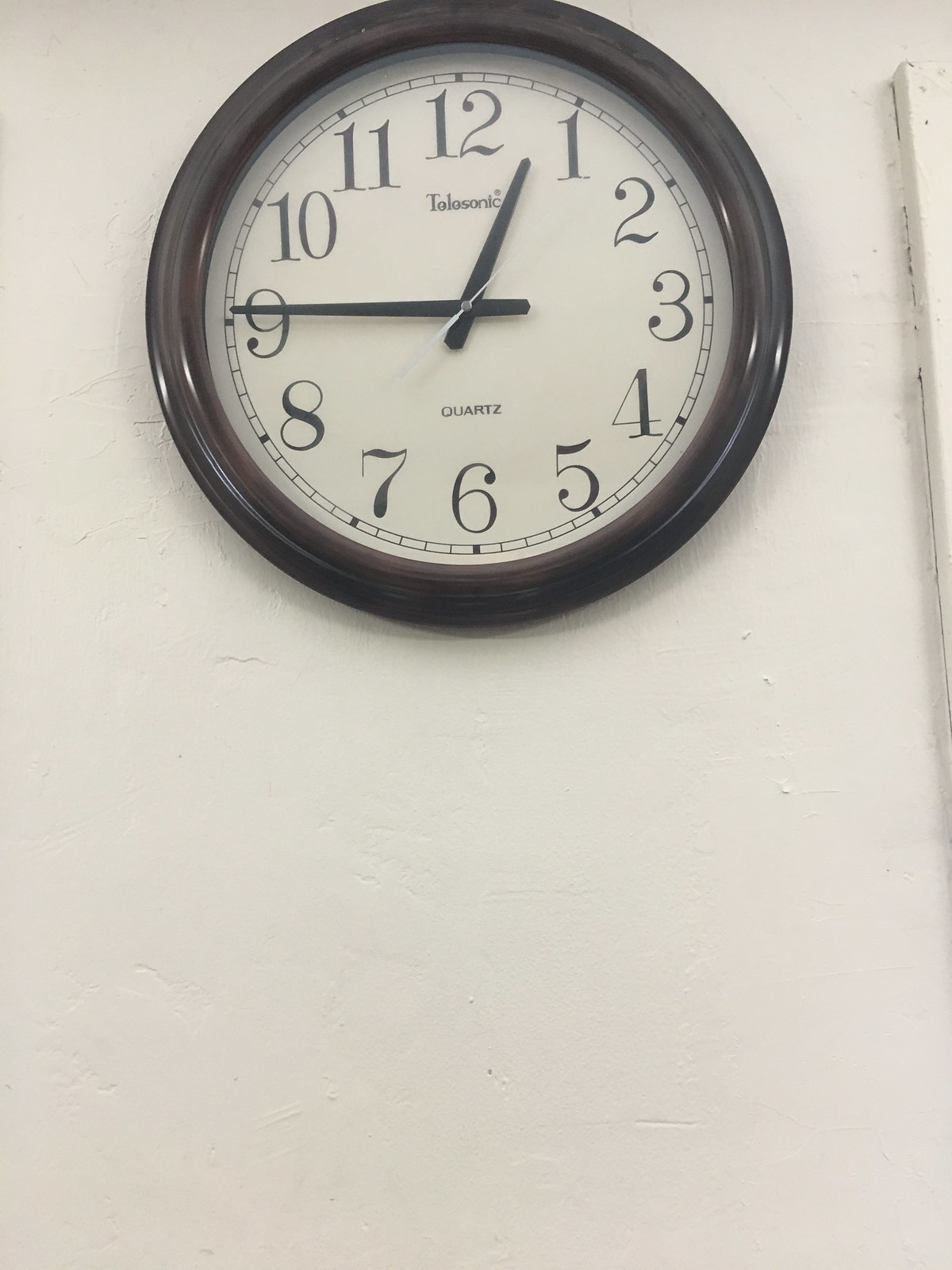The image is a detailed portrait-oriented color photograph focusing on a wall clock. The top of the photo prominently features the clock, slightly cut off at the top, revealing its dark brown walnut-effect bezel, possibly made of plastic. The clock's face is a beige, off-white cream color, contrasted by black hour and minute hands, and a white second hand. The time displayed is quarter to one, with the minute hand just past the 9 and the hour hand close to the 1. The white second hand is difficult to discern due to the image’s low resolution but appears to be between the 7 and 8. The clock has the brand name "TOLOSONIC" beneath the 12 and "QUARTZ" above the 6. The clock is mounted on a white plaster wall, which shows some rough spots and imperfections. Encroaching into the right side of the image is a door frame, slightly pulling away from the wall.